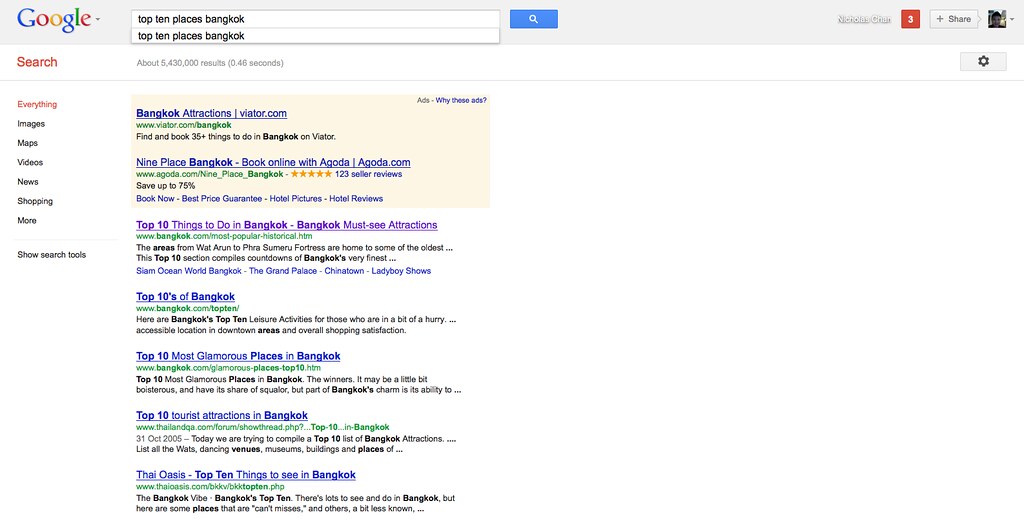Here is a cleaned-up and detailed description of the image:

---

This image is a screenshot of a Google search results page. At the top of the page, there is a light gray bar that spans the width of the screen. On the left side of this bar is the Google logo, which consists of the word "Google" with the letters colored in blue, red, yellow, blue, green, and red respectively. Next to the logo is a dropdown arrow. Below the gray bar, the search query "top ten places Bangkok" is visible in the search box, with "Bangkok" typed as "B-A-N-G-K-O-K". Next to the search box is a blue search button with a magnifying glass icon.

On the far right side of the top bar, there is a user's name, though it is difficult to discern. Alongside the name is a notification icon with the number three, a share button, and a small profile picture of a person with dark hair.

Beneath the search bar, the results information is displayed in red text, noting approximately "5,430,000 results in 0.46 seconds". To the right of this information is a "Settings" tab. Below, there are several navigation options: "All" (highlighted in red), "Images", "Maps", "Videos", "News", "Shopping", "More", and "Search tools".

The search results are displayed below these navigation options. The first result is from viator.com, titled "Bangkok Attractions - Viator" and includes a link to "Find and book 35 things to do in Bangkok on Viator". To the right of this entry is a label marked "Ad" with "Why these ads?" in a smaller font next to it.

The second result is "Nine Place Bangkok - Book Online" from agoda.com, featuring 123 seller reviews with a five-star rating.

The third result lists "Top Ten Things to Do in Bangkok" and highlights various areas, including "Wat Arun," "Phra Sumeru Fortress," among others.

The fourth result, from bangkok.com, is titled "Top Tens of Bangkok".

The fifth result is "Top Ten Most Glamorous Places in Bangkok," which includes a brief description.

The sixth result, titled "Top Ten Tourist Attractions in Bangkok," mentions the website and includes the date "31 Oct 2005".

The final result shown is "Thai Oasis - Top Ten Things to See" with additional descriptive text.

---

This caption accurately and thoroughly describes the various elements visible in the screenshot.